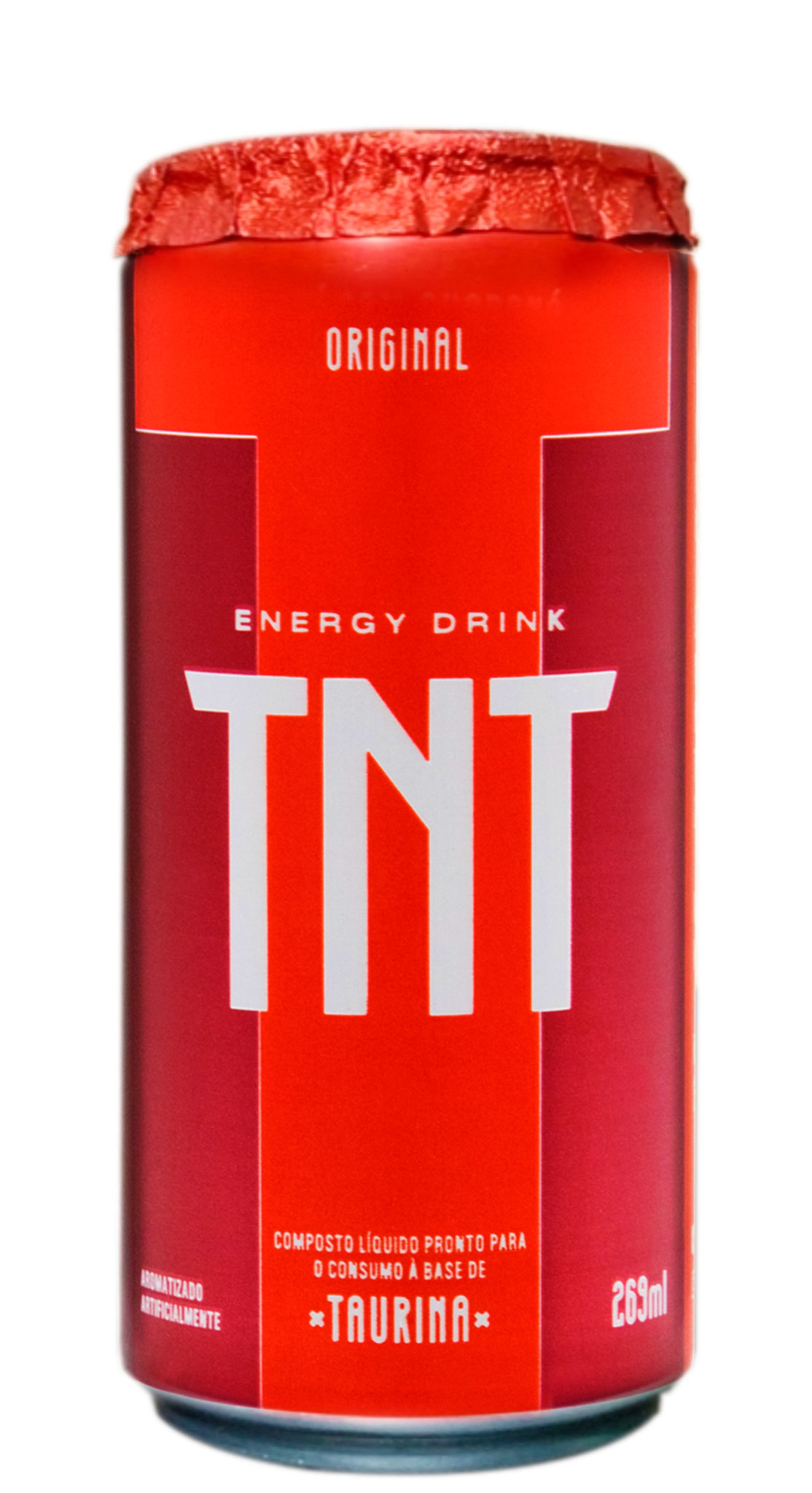The image depicts a tall, cylindrical can of the original TNT energy drink on a white background. The can is primarily cherry red with a deep red T-shaped design on the front, extending across the top and down the center. This T-shape is flanked by a darker, almost maroon red color. In white letters at the top of the T, the words "Original Energy Drink" are displayed, with "TNT" prominently printed in large letters below. The can's top is sealed with a red foil covering, pleated around the edges, instead of a traditional pull-tab. Additional details include a 269 ML marking in the bottom right corner, some small, unreadable text on the left, and Spanish words including "Torina" at the bottom center of the T-shaped area. The bottom of the can reveals its uncolored metal base. The text on the can also mentions "Composto Liquido Pronto Para o Consumo A base di Taurina" indicating its composition and readiness for consumption.